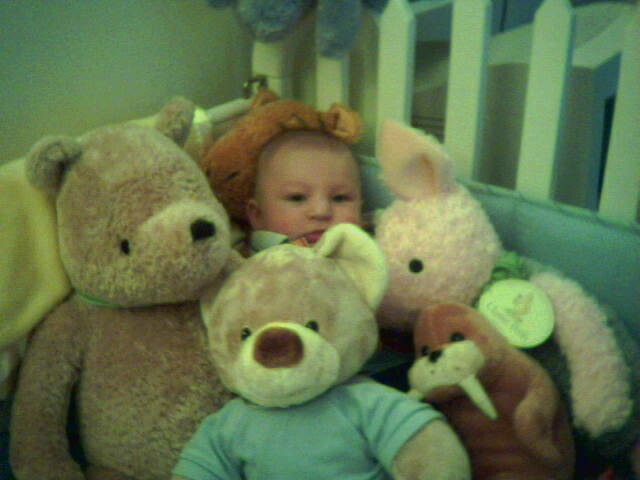This slightly blurry, low-resolution photograph captures a baby, approximately six months old, laying slightly propped up in the corner of what appears to be a crib, given the visible white slats toward the upper right and the surrounding padding. The infant, with sparse dark hair, gazes passively at the camera amidst an array of plush toys. To the baby’s left sits a brown teddy bear, while directly in front, another brown teddy bear wears a light blue t-shirt and has white fur around its muzzle. Positioned to the right are a walrus plush, identifiable by its two fangs, and above it, a pink pig stuffed animal. A white picket fence is seen behind the baby, alongside a green wall to the left, adding a quaint backdrop to this intimate scene.